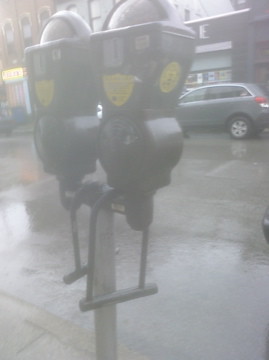The photograph is a blurry, portrait-oriented real-life image taken on a rainy city street, focusing on a double parking meter mounted on a single pole. The parking meters, gray and blue in color with circular tops and rectangular bodies tapering towards the base, feature a little silver coin slot and several yellow stickers. Two black U-shaped bike locks hang from the meters. The street and sidewalk appear slick from the rain, with visible wet surfaces. In the background, a gray car is parked in front of what resembles a mechanic's garage or gas station, and additional storefronts with multiple windows can be seen, though none are clearly identifiable due to the image quality. There are no people in the scene.